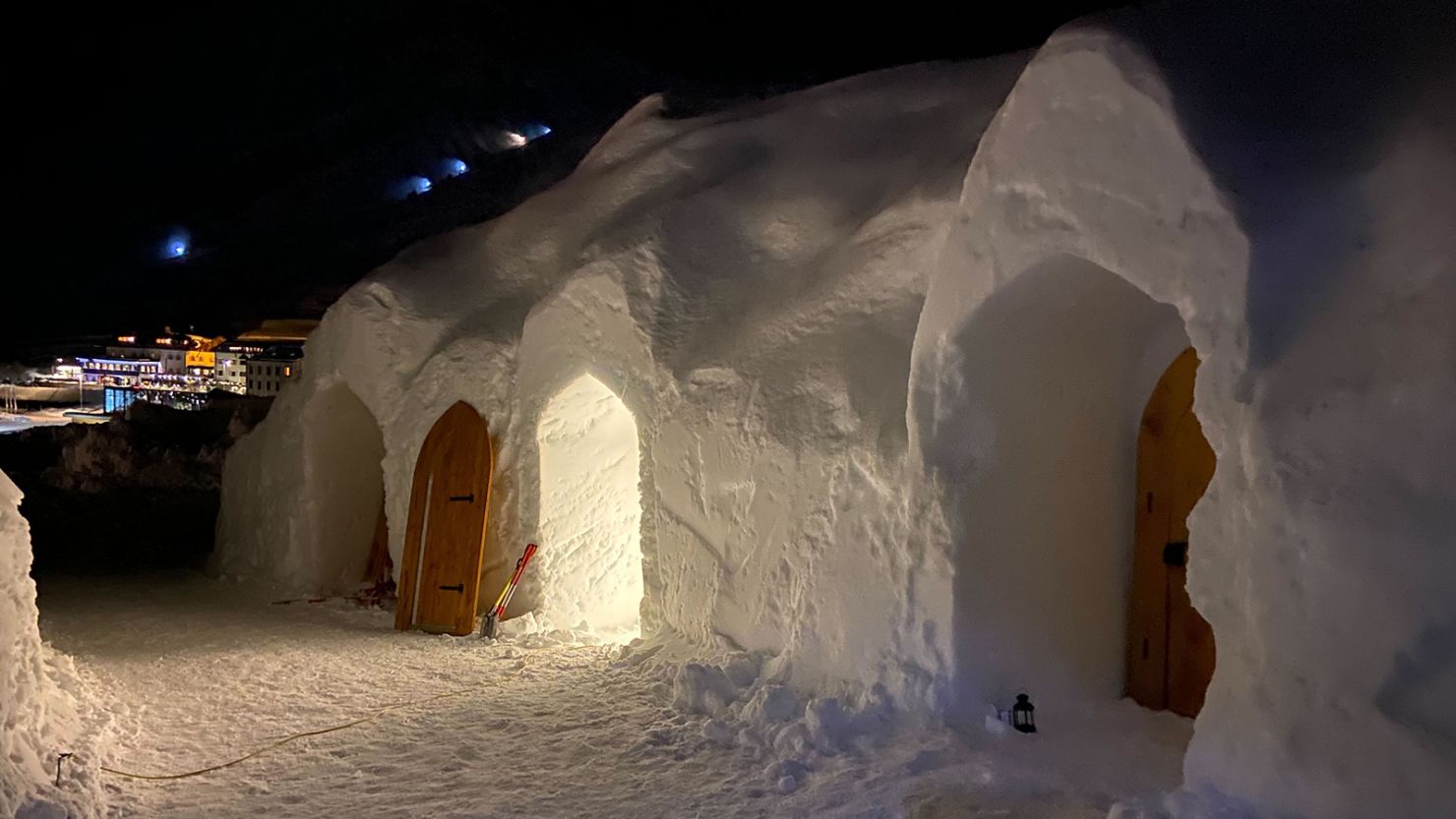In the photograph, a trio of igloos stand side-by-side in a snowy landscape under a dark, nighttime sky. The snow is well-trodden in front of each igloo, creating a clear walkway marked with footprints. The igloos, made entirely of packed snow, each feature wooden doors, with the entrance door of the middle igloo hanging off its hinge, allowing a warm light to escape from within. A wire can be seen running out from this same doorway. An unlit lantern sits in the entrance of the first igloo, casting a shadowy outline. In the distant background, there's an illuminated village with several buildings and taller structures, their lights twinkling against the night. Adding a touch of mystery, faint blue lights hover above the igloos, enhancing the serene and quiet ambiance of this unique, snowy habitat.